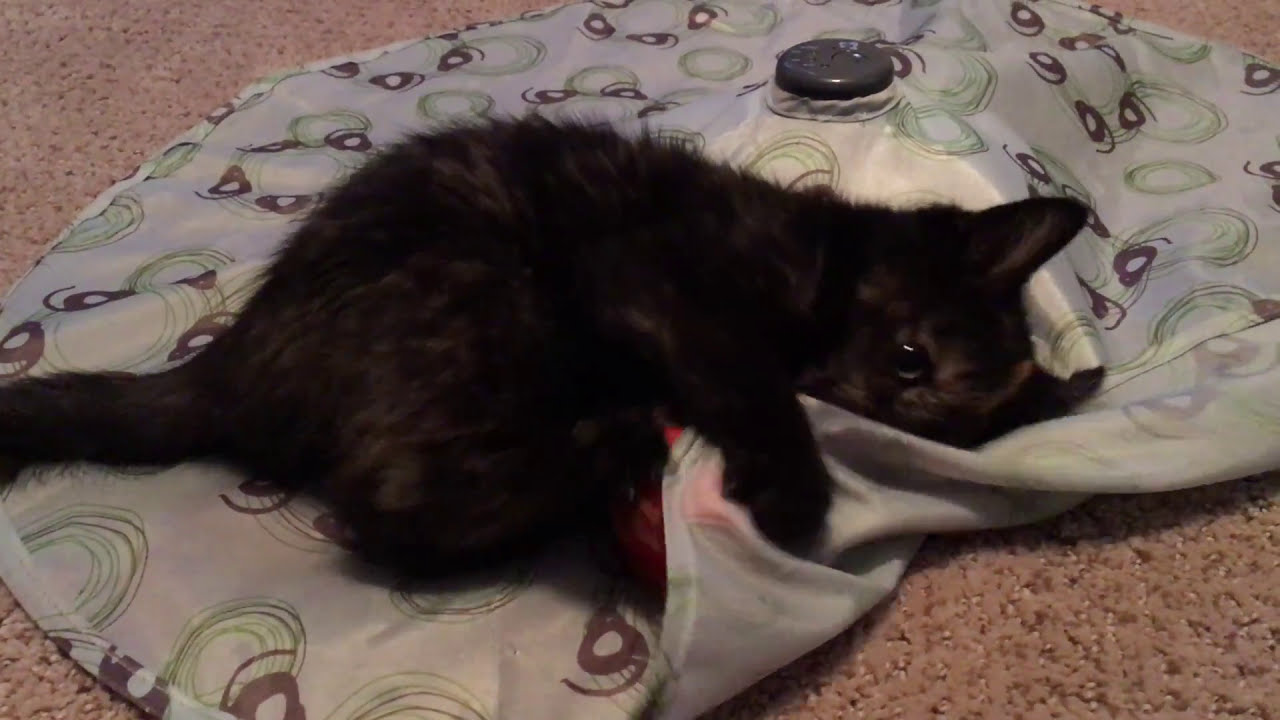A close-up image features a dark-colored kitten with light gray stripes, possibly a tortoiseshell pattern, lying on its side with one eye visible. The kitten is clutching a cloth with a geometric design consisting of green and brown circular patterns, almost as if embracing it. This material appears to be part of an inflatable object, possibly a bed or an inner tube, indicated by the visible gray air pressure seal located at the top center right of the image. The inflatable object has a grayish-purple and green swirly pattern and rests on a light brown, short-pile carpet. The kitten's tail extends beyond the left edge of the frame, adding to the cozy, intimate feel of the scene.